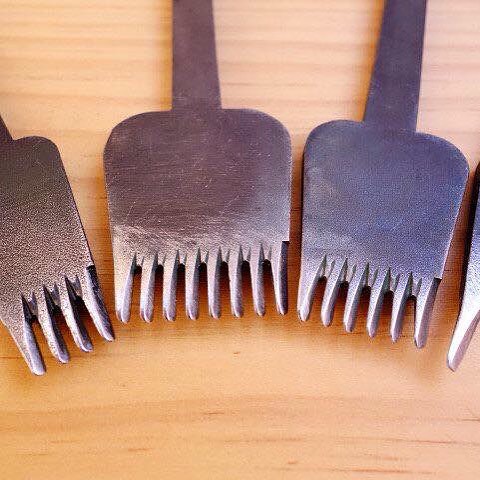This photograph captures four silver-gray metallic objects laid out on a light oak wooden table with visible wood grain. These objects resemble a combination of crude old forks and blades akin to barber clippers. They are crafted from solid metal with flat surfaces and have teeth-like prongs. Arranged in a semi-circle formation, the object on the left features four prongs. The first object in the middle is larger with eight prongs, while the second has six prongs. The fourth object is partially visible, showing only one prong. Each object's handle is flat, merging seamlessly with the rest of the structure, indicating they were likely cut from a single piece of metal. The prongs and flat metal surfaces suggest they could serve varied purposes, perhaps as short-tongued forks or portions of hair clippers.